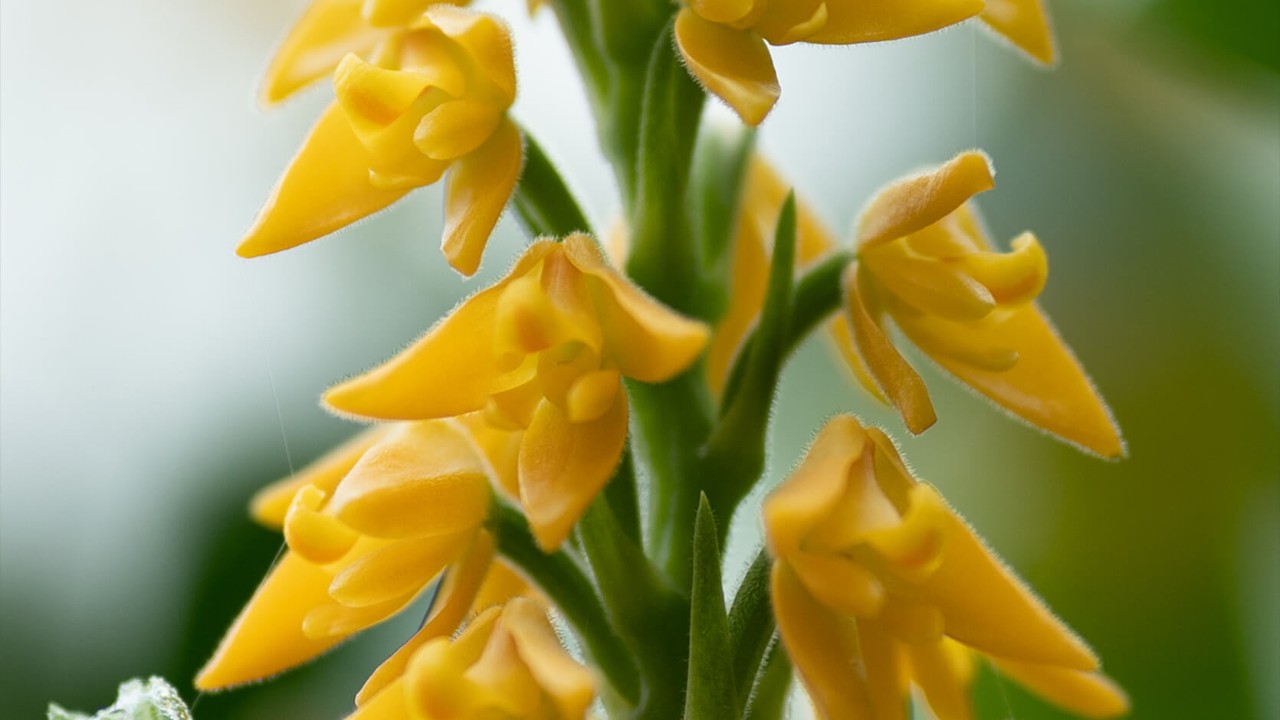This close-up nature photograph captures a striking Polystachia flower bud, showcasing its unique structure and vivid colors. At the heart of the image, a robust green stem emerges, adorned with fine hairs and branching into multiple smaller stems, each crowned with mustard-yellow petals. The composition reveals at least six distinct petals, all in sharp focus against a contrasting, blurred background. This out-of-focus backdrop melds white and green hues with hints of blue, enhancing the prominence of the flower. The petals, characterized by a mix of larger and smaller forms, exhibit the flower's intricate beauty. Additionally, a leaf reminiscent of an aloe vera plant contributes to the scene's complexity. The overall clarity of the flower and its vibrant yellow tones create a compelling focal point in this outdoor shot.